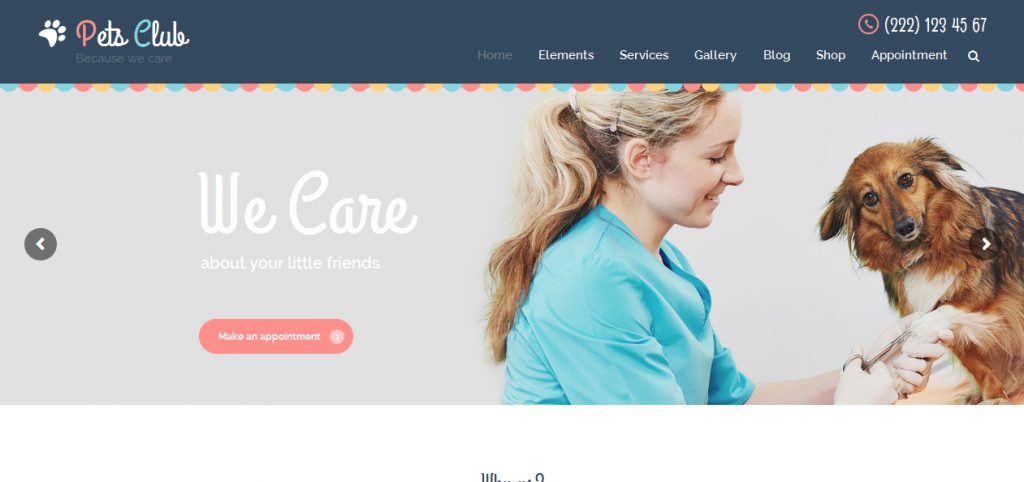This is a detailed caption for an image depicting an advertisement screenshot of the Pets Club website. 

"In this rectangular screenshot of the Pets Club website, the top left corner prominently features the company's name, 'Pets Club,' alongside their heartfelt slogan, 'Because We Care.' On the top right, there is a contact phone number clearly displayed as 222-123-4567. The website navigation menu, positioned just below the header, offers several options: Home, Elements, Services, Gallery, Blog, Shop, Appointment, and a search feature.

Central to the image is a photograph of a Caucasian woman with blonde hair, attentively grooming the nails of a beautiful dog. The dog appears well-cared for, with a striking coat in various shades of brown and a white chest. To the left of the grooming scene, there is a prominent call-to-action button inviting users to make an appointment. The overall design and layout of the screenshot are clean and easy to navigate, capturing the essence of Pets Club's dedication to pet care."